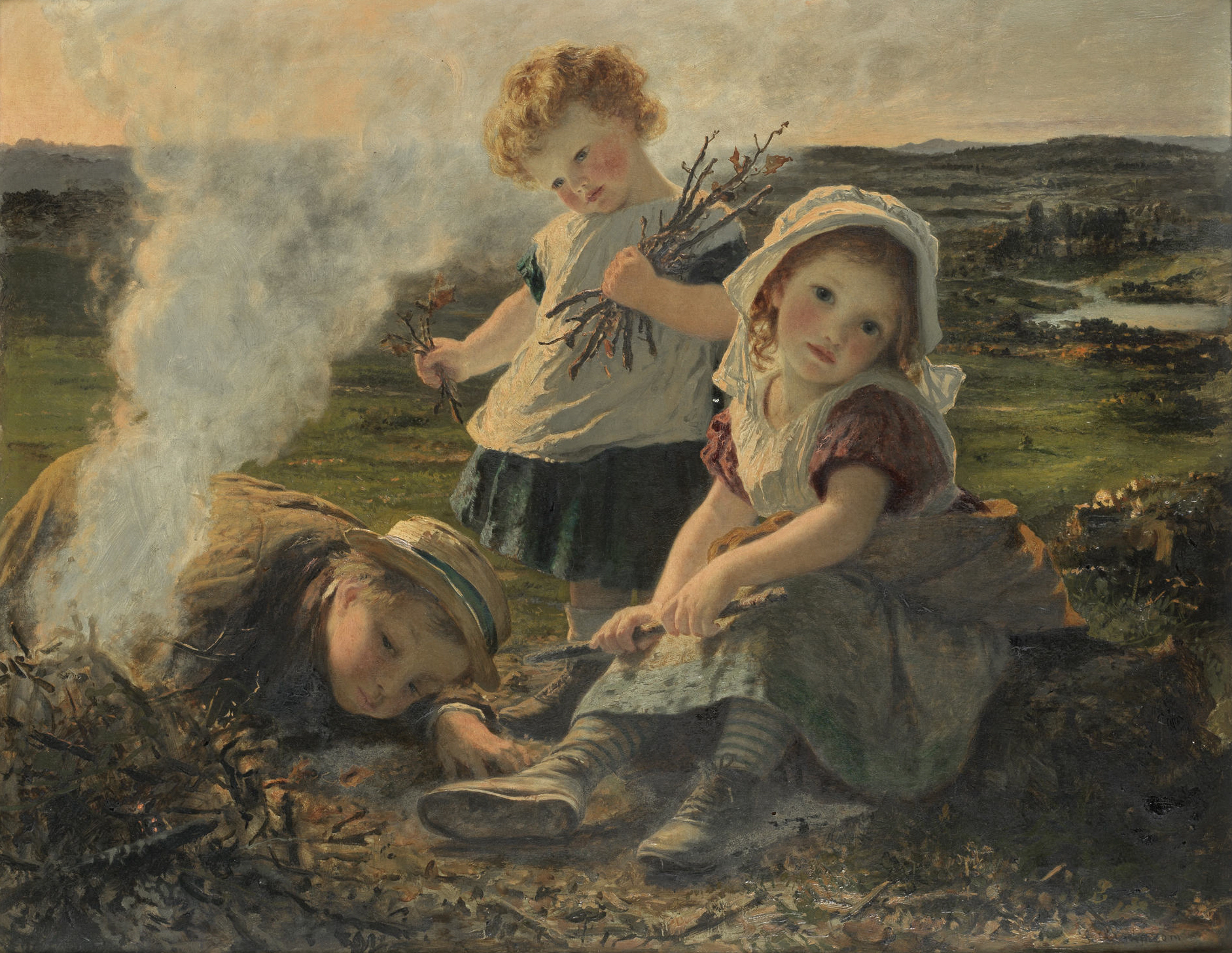The image is a detailed oil painting of three small children outdoors, gathered around a smoldering fire. Positioned at the lower left of the painting is a young boy with short blonde hair, wearing a straw hat with a blue band and a brown overcoat. He is lying on his stomach, intently observing the small fire made from a pile of twigs and leaves, which emits gray smoke. To the boy's right stands a young girl, around three years old, with short, curly, reddish-brown hair and rosy cheeks. She wears a white smock over a blue dress and holds a bundle of twigs against her chest with her left hand, holding a couple more sticks in her right hand. Seated to the right of this girl on either a rock or a log is another slightly older girl, around six years old, with similarly pale skin, rosy cheeks, and light reddish-brown curly hair. She wears a white prairie cap and a dress consisting of a white top with red puffy short sleeves and a grayish skirt. She has on striped socks and black shoes, and she holds a stick in each hand. Behind the children, the background reveals a green valley with rocky outcrops, a lake to the right, and a sky swirling with shades of gray and orange. The overall scene presents a nostalgic, serene moment captured in time.